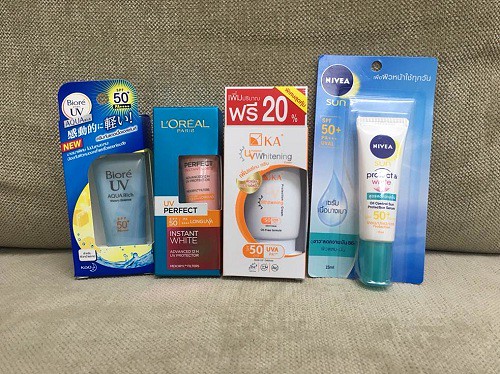A photograph captures an assortment of beauty products neatly arranged on a beige sofa with a heavy weave texture. The solid beige color of the sofa provides a neutral backdrop, highlighting the vibrancy of the packaged items. The beauty products, still sealed in their outer packaging, exude freshness and newness. Among the items, there's Biore UV in blue packaging, L'Oreal Perfect with blue, orange, and white hues, WS-20 in a simple white package, and Nivea Sun in light blue packaging adorned with a water drop design. All products feature tube packaging, ensuring a sleek and uniform appearance across the collection.